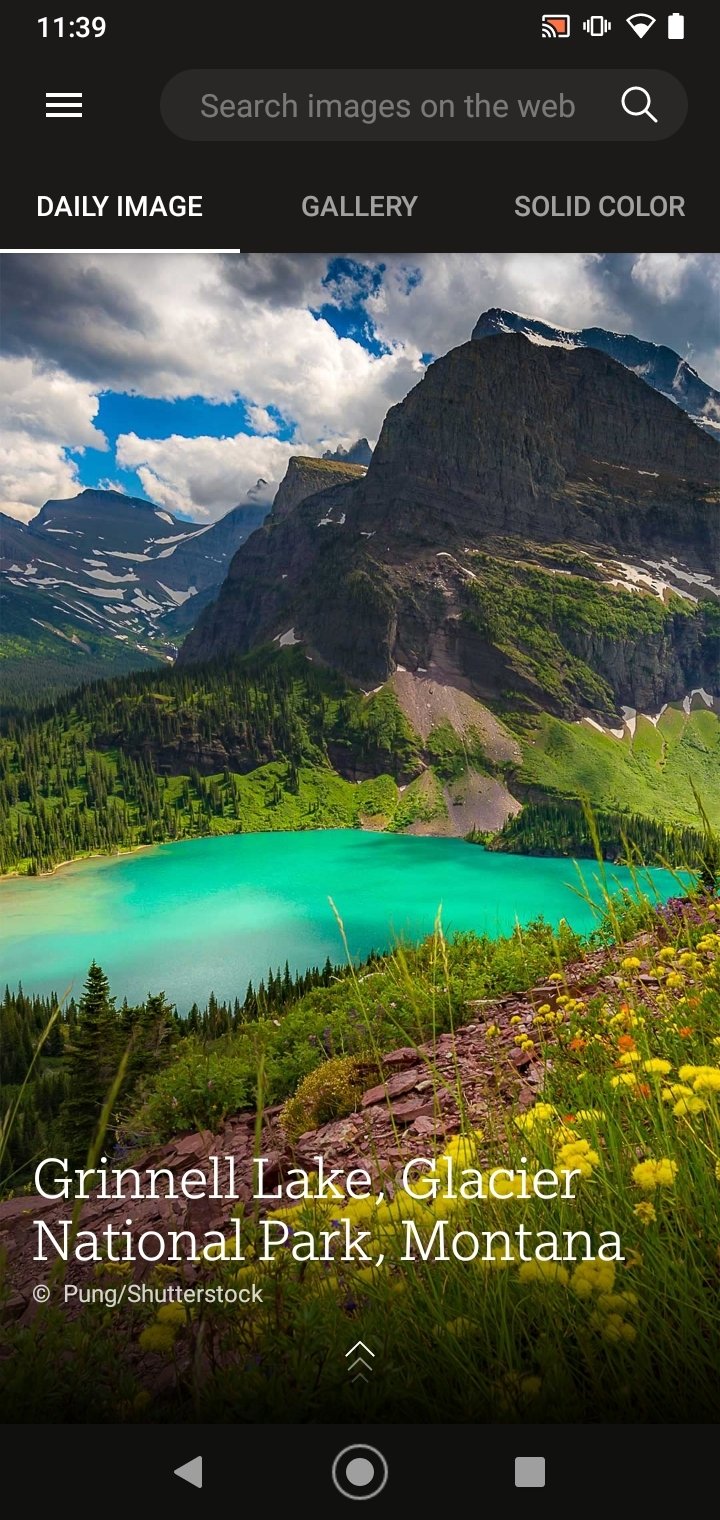The image captures the stunning Grinnell Lake in Glacier National Park, Montana. The lake's teal waters are accentuated with hints of white, likely from the reflection of the sky above. The sky itself is a vibrant blue, dotted with both white and a few gray clouds. In the distance, a range of majestic mountains looms, some still capped with patches of snow, particularly in shaded areas. Closer to the foreground, the landscape is lush with green grass and trees, interspersed with vibrant yellow flowers, primarily concentrated towards the right but extending towards the left of the frame as well. The white print on the image reads "Grinnell Lake, Glacier National Park, Montana" and denotes the copyright information from Pung Shutterstock. At the bottom of the image, there are symbols including a left-pointing triangle, a circle, and a square.